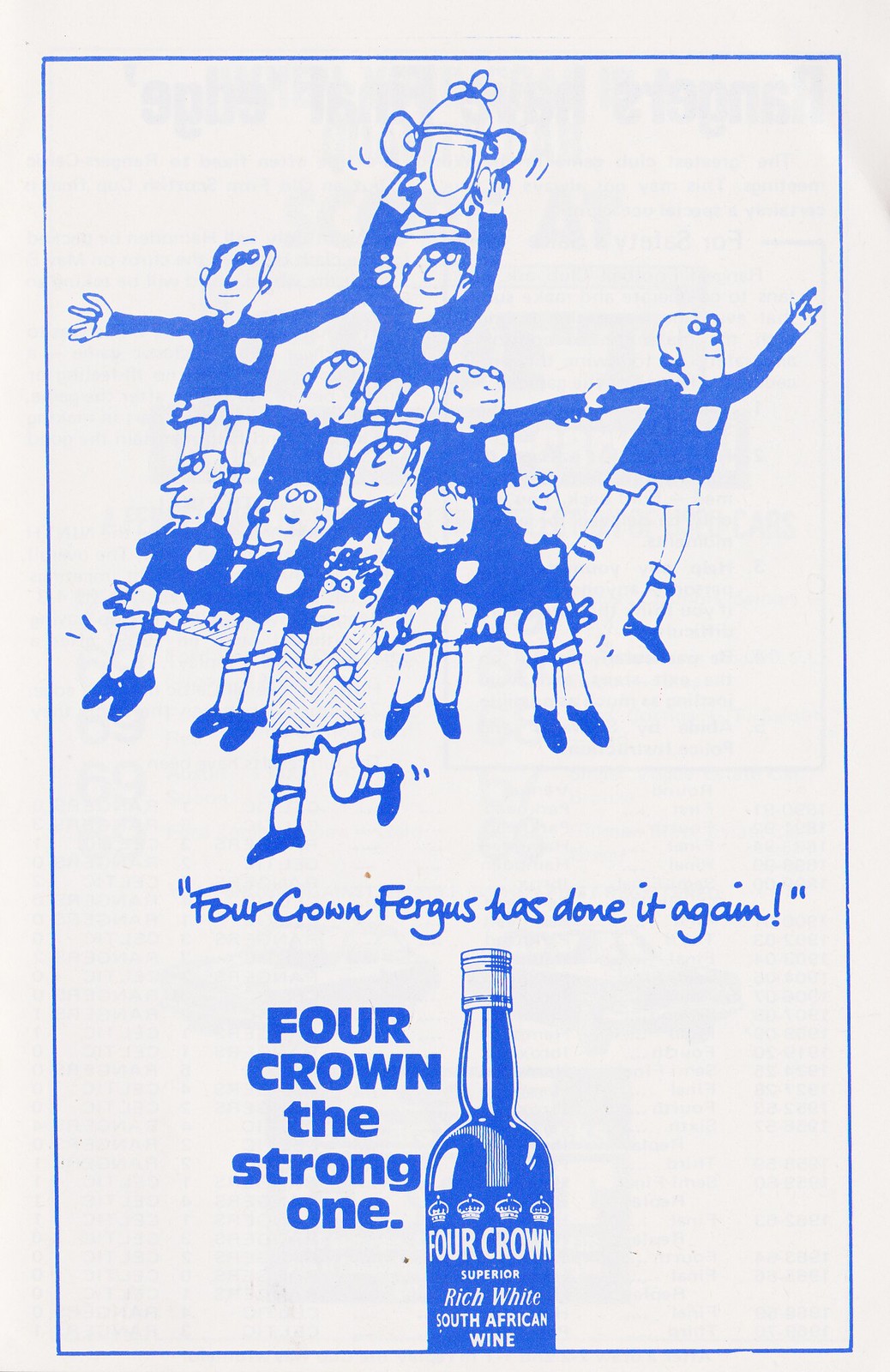This rectangular advertisement features a solid white background with bright blue elements. Central to the ad is an illustration in blue, depicting a man wearing a striped shirt and shorts, heroically holding up approximately ten soccer players. The soccer players, dressed in dark jerseys and striped socks, appear elated, with the player at the top proudly lifting a trophy. The scene exudes a vibrant energy of victory and joy. Beneath this illustration, the text in quotations reads "Four Crown Fergus has done it again." At the bottom, next to an illustration of a wine bottle, it states "Four Crown, the strong one." The bottle is labeled "Four Crown Superior Rich White South African Wine." All graphical elements and text follow the blue and white color scheme, complemented by a bold blue border.